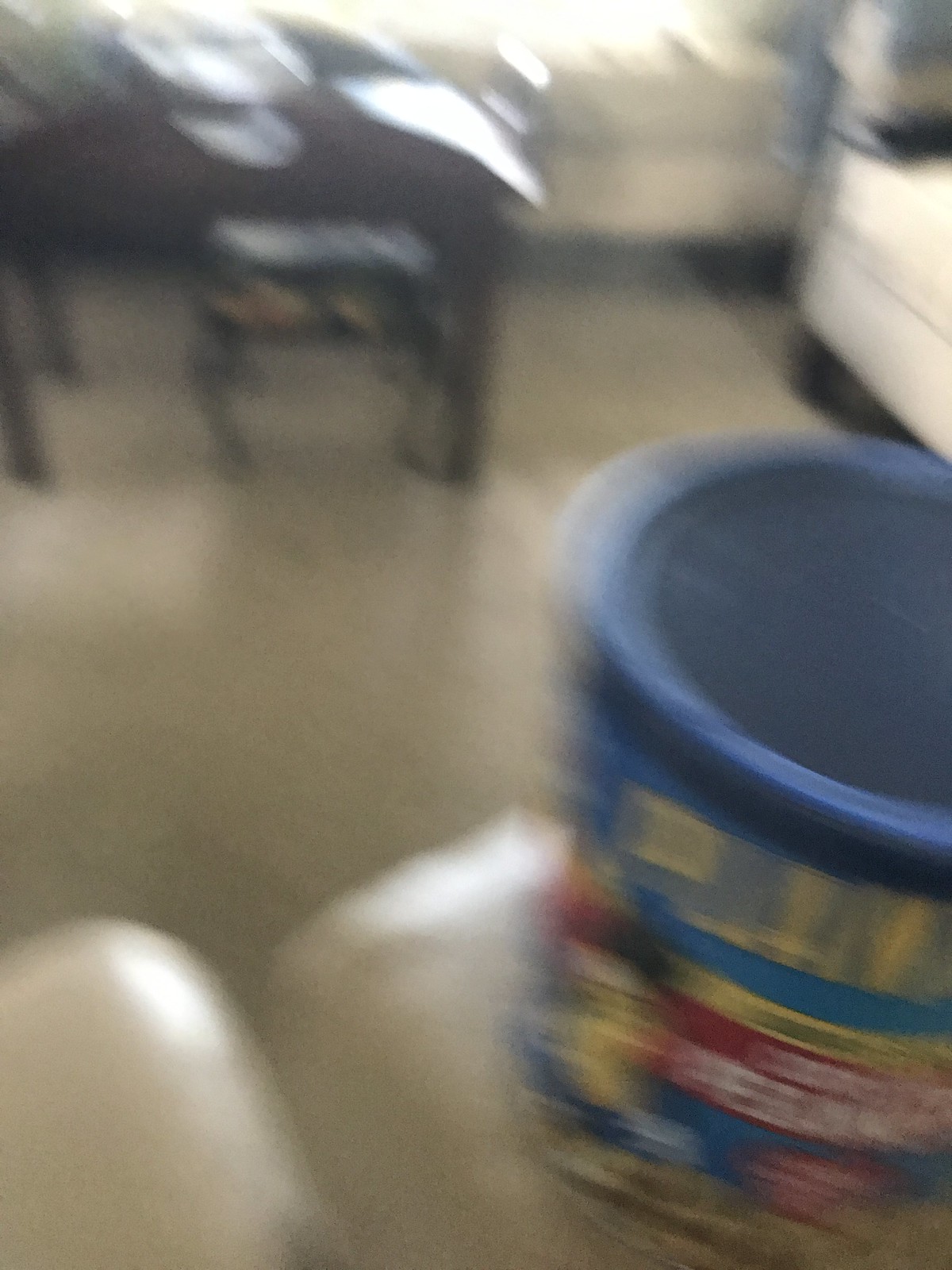This is a very blurry image depicting a living room. In the lower right-hand corner, there is a canister of Planters Peanuts with a blue lid, a yellow logo, and a red label featuring the iconic peanut character with a hat. The canister appears to be resting on the arm of a chair, and you can make out part of the individual's knee or leg nearby. The room features various furniture pieces, including a white couch with black legs to the far right, which is illuminated by light from a probable window behind it. In the vicinity, there is also a brown table and a white chair with brown legs. Draped over the white chair is a blue item, either a blanket or a shirt. The floor appears to be covered by a white rug, and there are multiple pieces of furniture scattered around, such as additional leather couches or chairs.